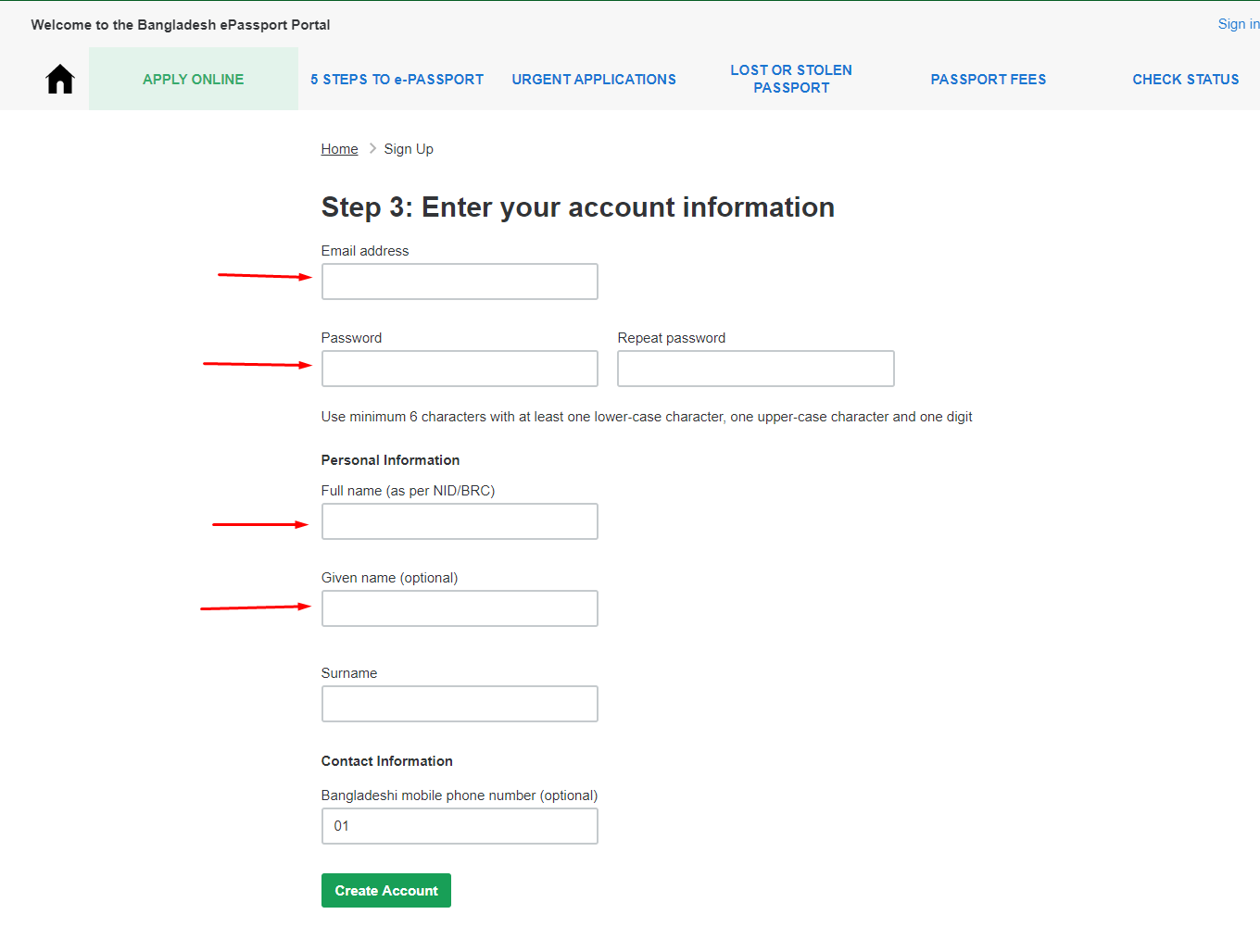The image showcases the Bangladesh e-passport portal, an online platform for applying for an e-passport. The central portion of the portal features fields for entering essential information such as name, address, and other personal details. To assist users in correctly filling out the application, red arrows are prominently displayed, highlighting where specific information should be entered. Additionally, the "Apply" button is visibly marked in green, guiding applicants on how to submit their completed forms. The overall layout is user-friendly, designed to make the application process straightforward and accessible.